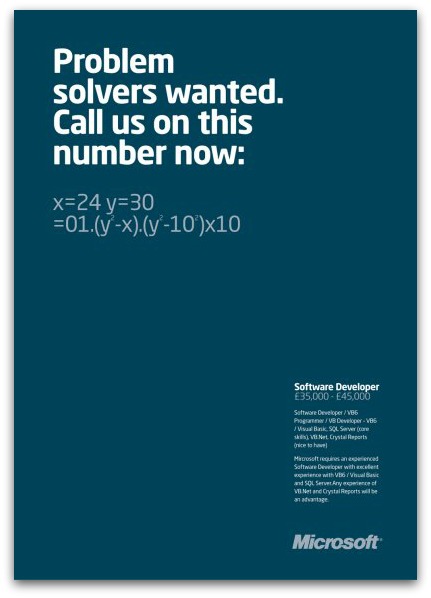The image features a solid dark blue background with white text. In the top left corner, bold letters read "Problem Solvers Wanted." This is followed by the prompt "Call us on this number now." Directly beneath, there is a mathematical equation: "X = 24, Y = 30, 0.1(Y^2 - X)(Y^2 - 10^2) * 10."

In the bottom right corner, it states "Software Developer" and indicates a salary range of "£35,000 to £45,000" (the previous mention of euros was incorrect). Below this, the text reads "Software Developer / VB6 Programmer / VB Developer - VB6 - World Bank - SQL Server." Further details include: "Microsoft requires an experienced software developer with excellent experience in VB and SQL Server. Experience with .NET and Crystal Reports will be an advantage." 

At the very bottom, the name "Microsoft" is visible, written in a subtle but readable manner.